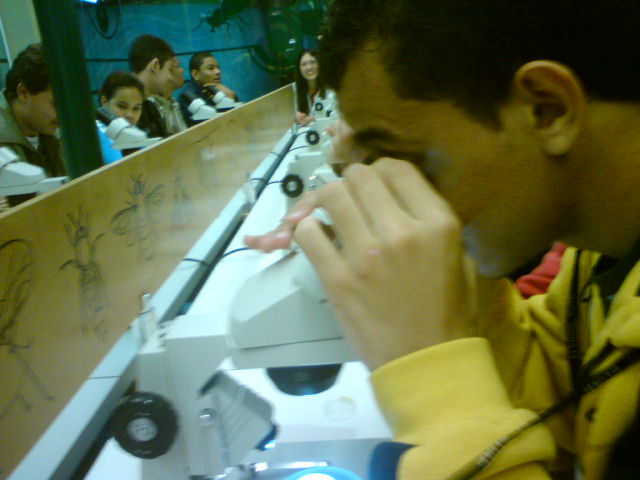In this detailed, color horizontal photograph, we see a man with dark hair and very short hair wearing a yellow jacket and a black lanyard around his neck, intently looking through a cream-colored microscope with both his hands gently holding it. The microscope is illuminated at the base where the specimen would sit. This photo, likely taken with a personal camera indoors in a setting that resembles a museum, captures a scene filled with other individuals, both male and female, engrossed in their own observations through identical microscopes lined up on a long table.

A brown divider runs down the middle of the table, adorned with detailed drawings of various insects, each positioned in front of a microscope. Directly behind this divider and at the table's far end sits a woman with long black hair, wearing a white jacket and smiling, not currently engaged with a microscope. The surrounding people, who all appear to have dark hair, are deeply focused on what they are viewing. The backdrop of the scene includes a blue wall. The overall atmosphere suggests a shared, immersive educational experience.